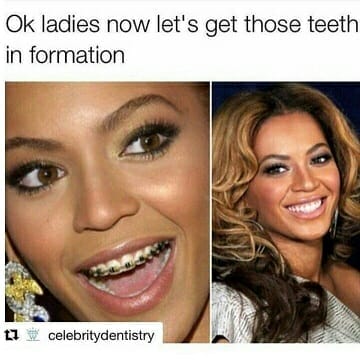The image is a promotional material, likely a tweet, showcasing the dental transformation of an African-American woman, identified as Beyoncé, through orthodontic work. The top of the image features the text, "Okay ladies, now let's get those teeth in formation," in black. Below this, there are two side-by-side photos. The left photo is an extreme close-up of Beyoncé smiling with her mouth open, revealing metal braces on her teeth. In the right photo, a slightly more distant shot, Beyoncé is smiling broadly without braces, her straight, white teeth on display. Her brown eyes and light brown hair, parted in the middle and styled in big curls cascading past her shoulders, are especially noticeable in this picture. The bottom of the image contains the text "celebrity dentistry."